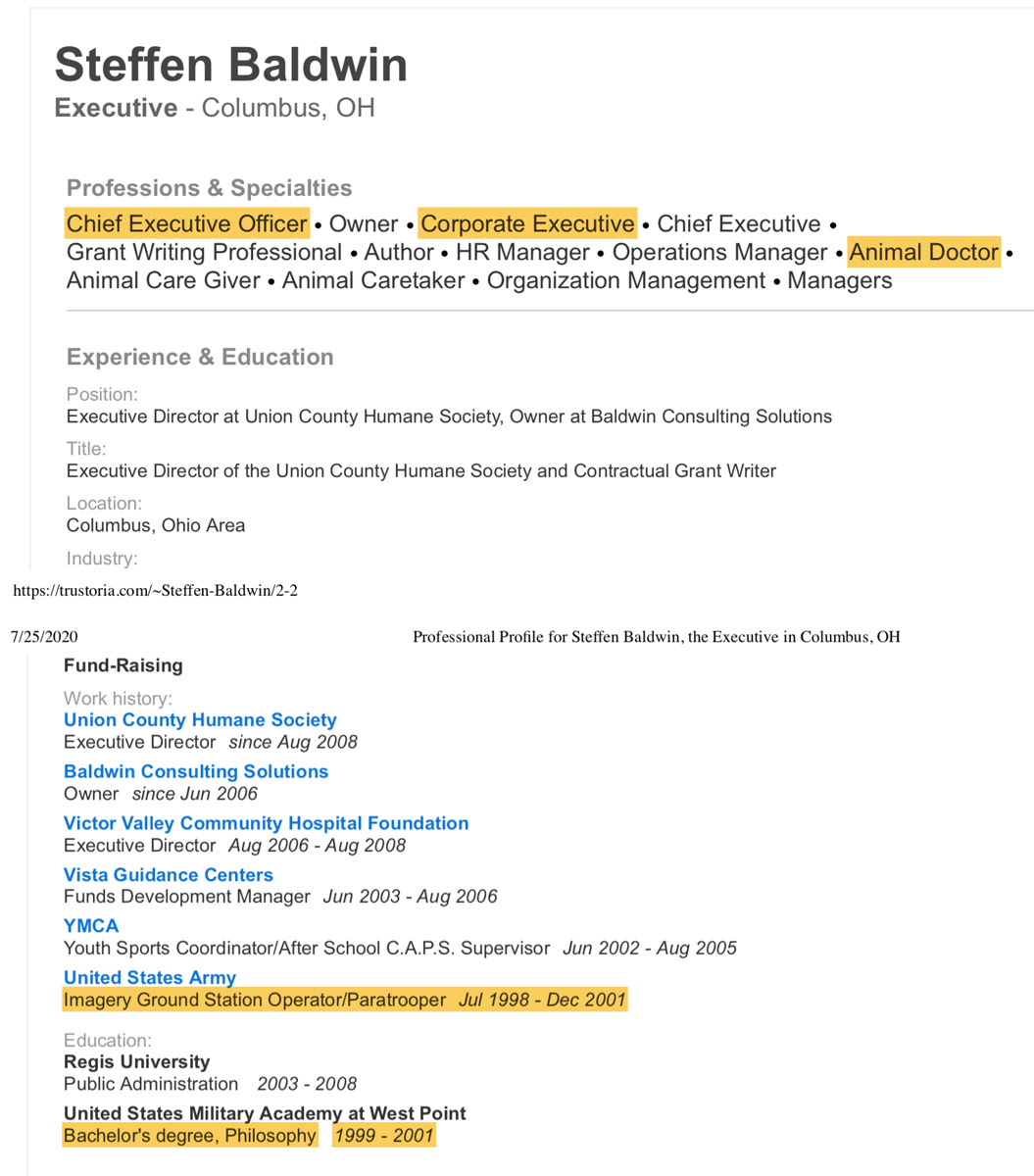**Profile Summary of Stephan Baldwin**

---

**Header:**

*Stephan Baldwin*

- **Location:** Columbus, Ohio
- **Position:** Executive Director
- **Industry:** Organization Management

---

**Profession and Specialties:**

1. Chief Executive Officer (Highlighted in orange)
2. Owner
3. Corporate Executive (Highlighted in orange)
4. Chief Executive
5. Writing Professional
6. Author
7. HR Manager
8. Operations Manager
9. Animal Doctor (Highlighted in orange)
10. Animal Caregiver
11. Animal Caretaker
12. Organization Management
13. Manager

---

**Experience and Education:**

- **Current Positions:**
  - Executive Director at Union County Humane Society
  - Owner at Baldwin Consulting Solutions
  
- **Titles:**
  - Executive Director of the Union County Humane Society
  - Contractual Grant Writer

- **Work History:**
  1. Union County Humane Society (Executive Director since August 2008)
  2. Baldwin Consulting Solutions (Owner since June 20, 2006)
  3. Victor Valley Community Hospital Foundation (Executive Director from August 2006 to August 2008)
  4. Vista Guidance Centers (Funds Development Manager from June 2003 to August 2006)
  5. YMCA (Youth Sports Coordinator / After School CAPS Supervisor from June 2002 to August 2005)
  6. United States Army (Imagery Ground Station Operator / Paratrooper from July 1998 to December 2001)

- **Education:**
  - **Utah State University:** Public Administration (2003-2008)
  - **United States Military Academy at West Point:** Bachelor's Degree in Philosophy (1999-2001)

---

**Industry Resource:**

- For more detailed information, visit: [https://trustorio.com/Stephan-Baldwin-2-2](https://trustorio.com/Stephan-Baldwin-2-2)

---

**Professional Profile Overview:**

*Stephan Baldwin,* a seasoned executive based in Columbus, OH, possesses extensive experience in fundraising and organizational management. His professional journey is marked by significant roles, ranging from Executive Director positions to owning consulting solutions and leading animal care organizations. Stephen’s comprehensive career spans both the non-profit sector and military service, highlighting his diverse expertise and dedication to leadership and community service.